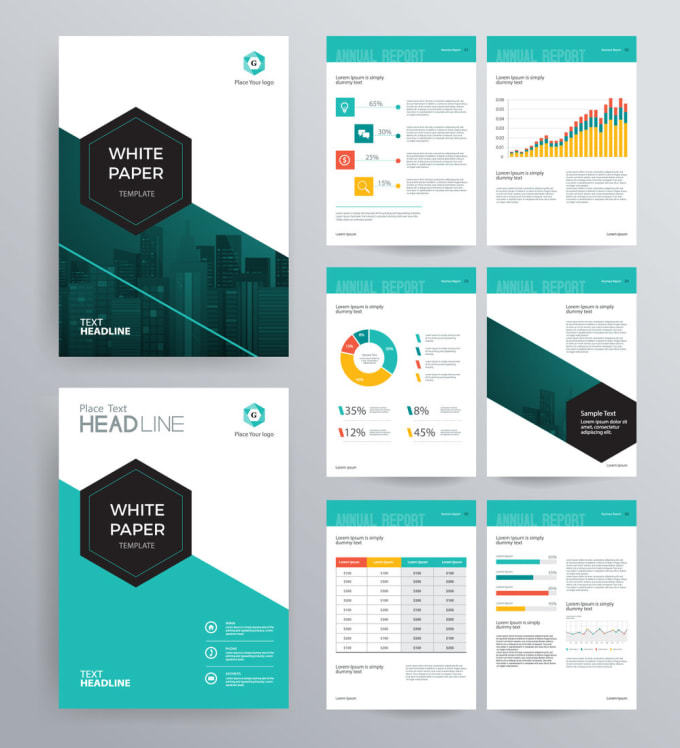The image is a detailed advertisement for a white copy paper template, designed for creating annual reports or similar documents. On the left side, there are two prominent images labeled as "white paper template", one encircled with a black hexagon, intended for users to place their logo and text headline. A prompt suggests placing the text headline or logo, hinting at customization. The background has a light gray tone, enhancing the visibility of the content.

On the right side, there are six smaller images showcasing different sections of what appears to be a well-structured annual report or instruction manual. These sections display a variety of graphical representations including bar graphs, circular charts, pie charts, and lists. The charts feature color coding in blue, dark blue, red, yellow, green, and more, implying a rich design capability. Each template section is sample-labeled with placeholder text that’s too small to read clearly, emphasizing its customizable nature rather than being a final product. 

The charts and graphs are also set against a clean background, with some layouts divided diagonally into blue and white segments to indicate their structure. Overall, the advertisement effectively illustrates the versatility and professional quality of the copy paper templates, suggesting they are ideal for designing and presenting detailed and colorful reports.